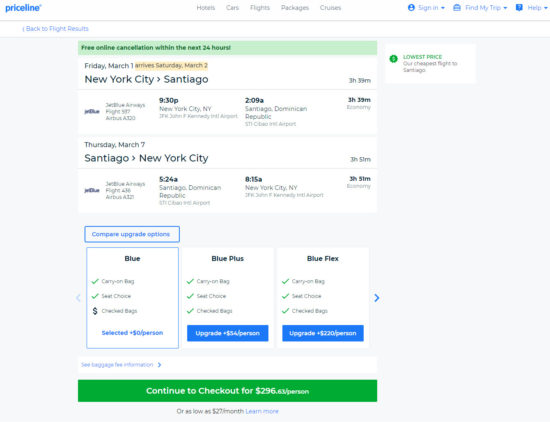The webpage displays a Priceline booking interface, prominently featuring their logo in the upper left corner against a white background. The logo is blue, creating a striking contrast.

Moving towards the center of the screen, a gray navigation bar offers various options including "Home," "Hotels," "Cars," "Flights," "Packages," and "Cruises." On the right side of the navigation bar, there are several interactive elements: a "Sign In" button with a drop-down menu, "Find My Trips" with another drop-down menu, and a "Help" option, also with a drop-down menu.

Below the navigation bar, the webpage indicates "Back to Flight Results" in a clear font. Centered on the page, there is a green banner with darker green lettering, informing users about "Free Online Cancellation within the Next 24 Hours."

Directly beneath this banner, on a white background, there's detailed flight information. The departure details are as follows:
- **Departure:** Friday, March 1st
- **Arrival:** Saturday, March 2nd
- **Route:** New York City (JFK) to Santiago, Dominican Republic (STI)
- **Duration:** 3 hours and 33 minutes
- **Class:** Economy

A grey line separates the next section, detailing flight times:
- **Departure Time:** 9:30 PM from New York City (JFK)
- **Arrival Time:** 2:09 AM in Santiago, Dominican Republic (STI)

The resolution of the image is poor, making it difficult to read some of the text. However, the return flight details are partially visible:
- **Return Flight:** Thursday, March 7th
- **Route:** Santiago, Dominican Republic (STI) to New York City (JFK)
- **Duration:** 3 hours and 51 minutes
- **Class:** Economy
- **Departure Time:** 5:24 AM from Santiago
- **Arrival Time:** 8:15 AM in New York City

The image captures the essential travel information but is hindered by low resolution, making some details challenging to discern.